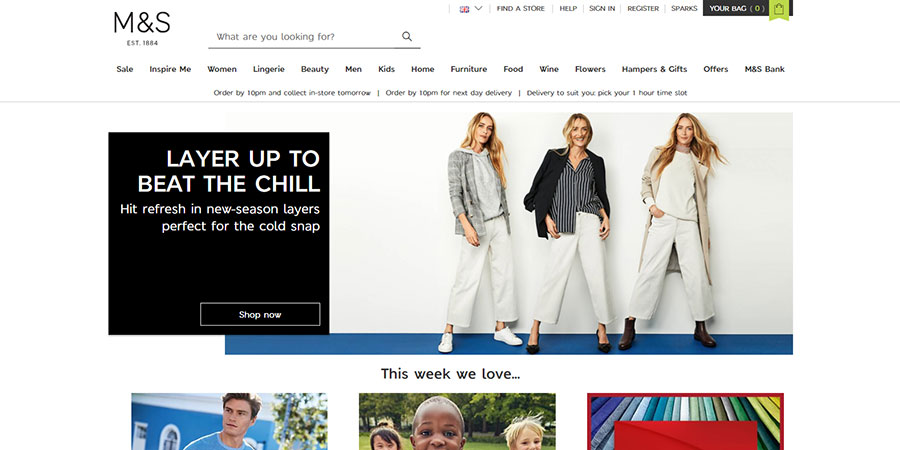**Caption:**

The image showcases the homepage of the M&S shopping website, characterized by a clean white background. Positioned at the top left corner is the brand logo that reads "M&S", followed by the tagline "Established 1984". To the right of the logo is a compact search bar for easy navigation of products. Adjacent to the search bar is a small icon representing the main menu. 

On the right-hand side of the header, options for changing the country of purchase are displayed first. Following this are links for "Find a Store," "Help," "Sign In," "Register," and "Sparks," with the extreme right featuring the "Add to Cart" or "Bag" icon.

Beneath the header, a detailed navigation menu spans across the page, listing categories such as Sale, Inspire Me, Women, Lingerie, Beauty, Men, Kids, Home, Furniture, Food, Wine, Flowers, Hampers and Gifts, Offers, and M&S Bank.

Directly below this menu are three concise service messages: "Order by 10 p.m. and collect in-store tomorrow," "Order by 10 p.m. for next day delivery," and "Delivery to suit you: Pick your one-hour time slot."

The central area of the page features an image of a woman modeling three different semi-casual outfits. The first outfit consists of grey pants, a white shirt, a grey hoodie, and a blazer. The second outfit maintains the same pants but pairs them with a striped black top and a black blazer. The third ensemble again uses the same pants, complemented this time by a white sweatshirt and a long trench coat.

Below this central image are three somewhat cropped images; the first appears to feature a man in a blue top or shirt, and the second shows children. The third image is not fully visible.